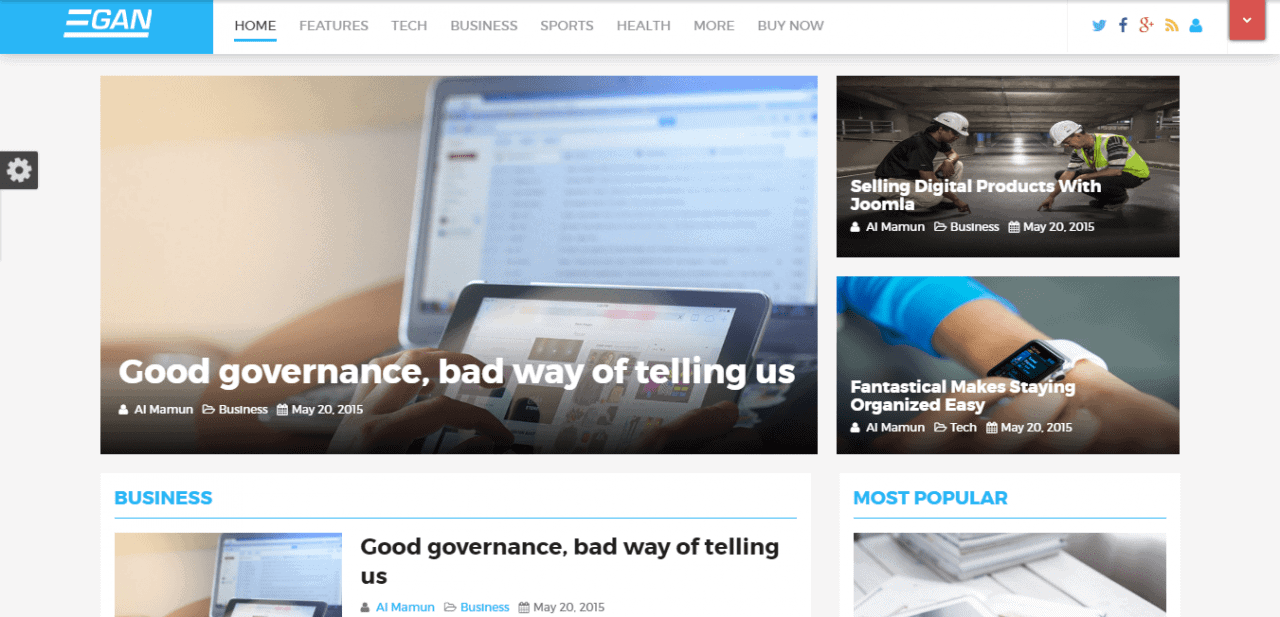In the upper left corner, the image features a baby blue background with white text that reads "Gain" in large font. Below, in black text, the word "Home" is highlighted with a blue underline. Subtitles in gray list various categories: "Features," "Tech," "Business," "Sports," "Health," and "More." Moving to the right, icons for social media platforms are displayed, including Twitter, Facebook, Gmail, and Google Plus, along with a full Wi-Fi signal icon, a profile picture of a person, and a black box containing a white drop-down arrow.

The main background of the image is gray, with a black gear icon located on the right-hand side. Surrounding the gear icon are a variety of smaller photos. One photo shows an individual using a laptop, another depicts someone holding a tablet, presumably with an open email application, and a white hand interacting with the tablet screen. 

White text overlaid on the photos reads: "Good Governance, Bad Way of Telling" and below it "Al Mommy Business, May 20, 2015." To the far right, a smaller image displays two individuals wearing white hard hats inside a building under construction; one of them is wearing a yellow work vest. Additional text indicates this story is about "Selling Digital Powers with Juma," authored by the same person on the same date. 

Lastly, the bottom section repeats the "Good Governance, Bad Way of Telling" theme, with another entry showing someone looking at a smartwatch. This part states: "Tech, May 20, 2015," tying back to the consistent author and date. The image encapsulates a well-rounded blend of tech news, business updates, and social media interactions reflecting the publication's multifaceted content.